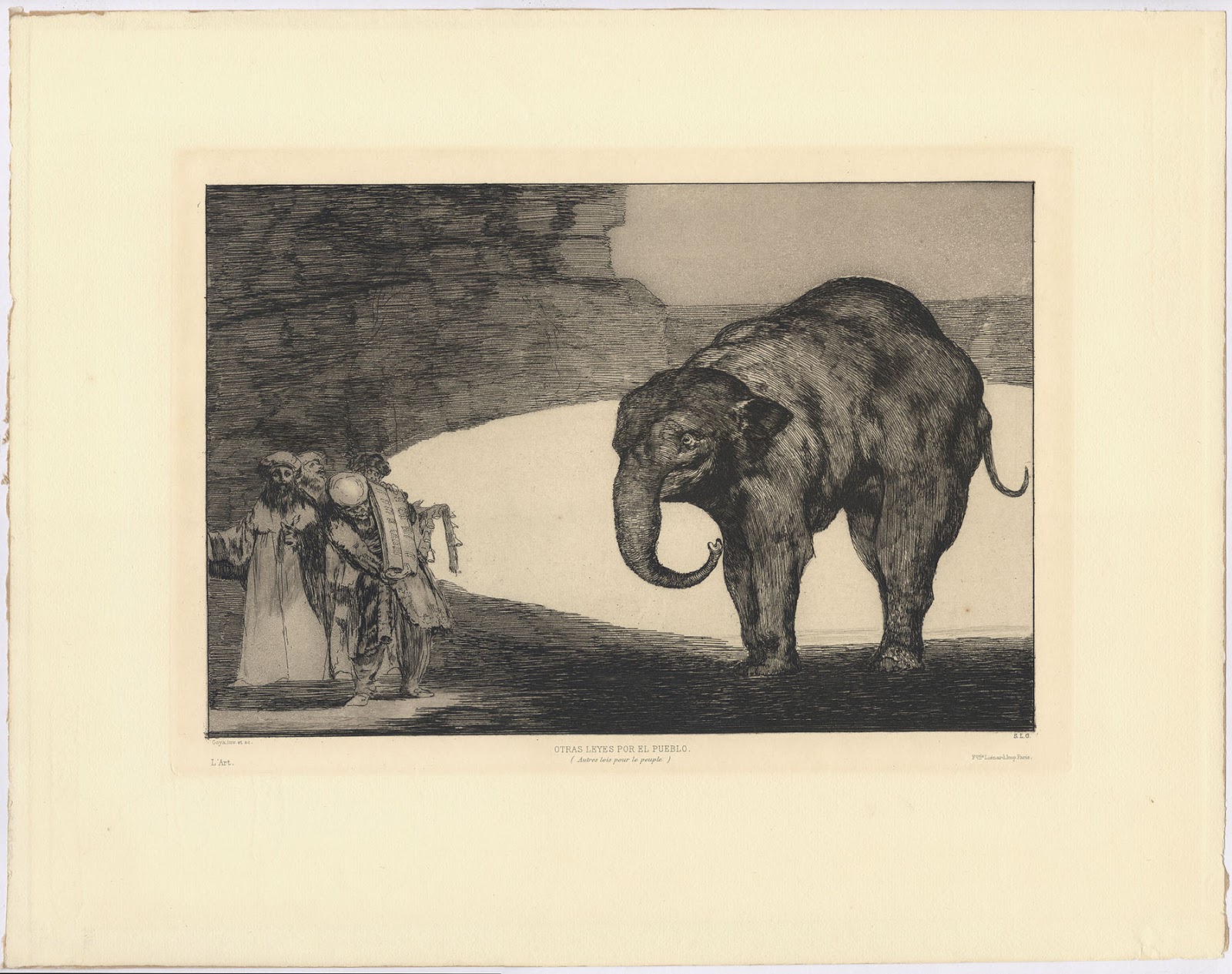This is a detailed scan of a horizontal, rectangular pen and ink drawing, mounted on a yellowed backing, giving it an aged appearance. The artwork features a muscular, unique-looking elephant with a bumpy texture, small ears, a trunk curved underneath it, and a tail curved over its back, standing in a body of water. To the far left, there are two to four robed men with beards, possibly carrying a blanket, wading through the water. Behind them is a large stone cliff or rock formation, with a darkened sky visible over the scene. The background stretches to show water in the far distance. There are inscriptions beneath the elephant, likely the name of the artwork and the artist, but they're too small to discern. The image has a yellow border, enhancing its antique feel.